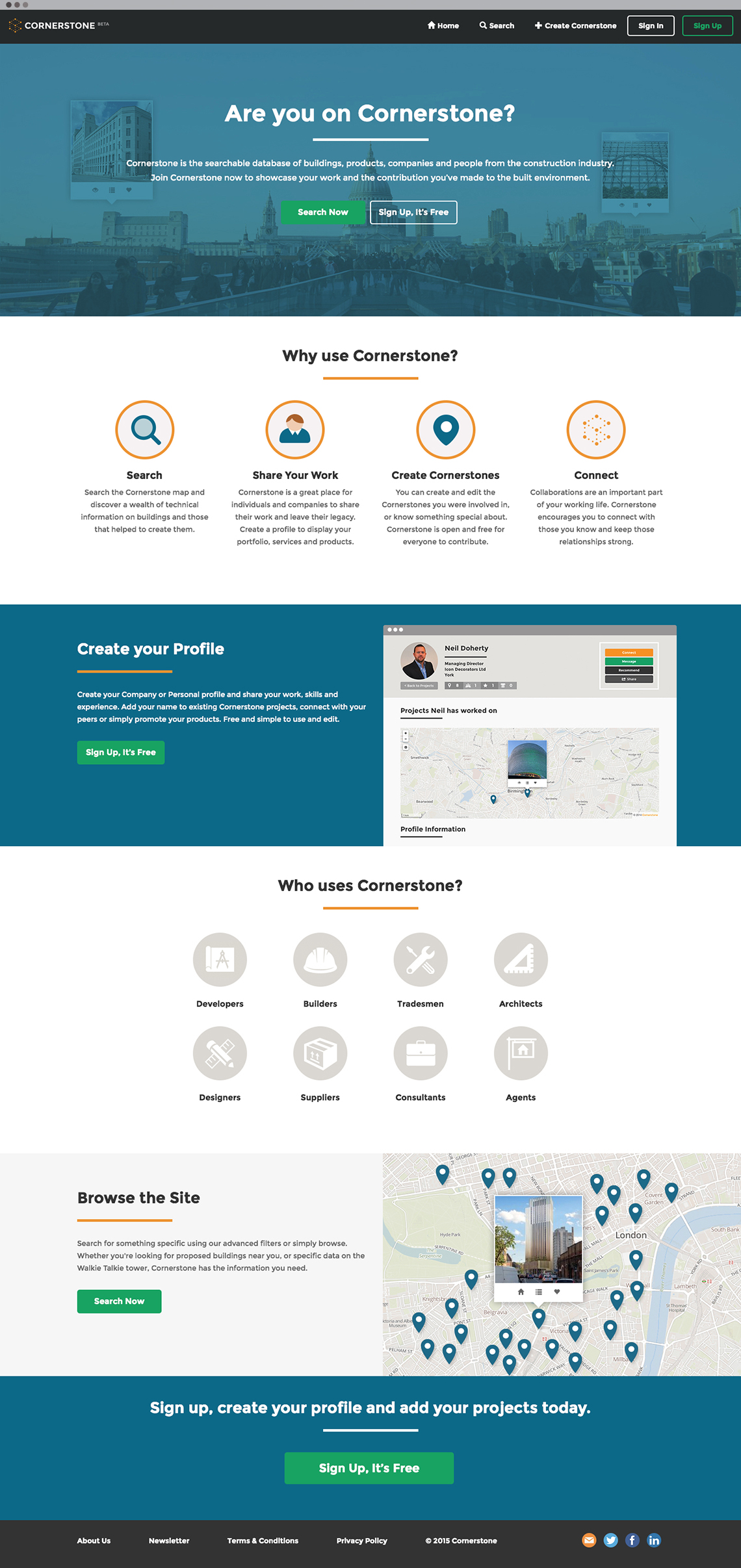The top section of the webpage features a striking black background with the word "Cornerstone" prominently displayed in white text. Adjacent to this are navigation options: "Home," "Search," "Create Cornerstone," followed by "Sign In" in white and "Sign Up" in green to draw attention.

A detailed cityscape serves as a backdrop, infusing the page with an urban ambiance. In white text, a headline asks, "Are you on Cornerstone?", underlined for emphasis. Below this, the site description reads: "Cornerstone is a searchable database of buildings, common products, companies, and people from the construction industry. Join Cornerstone now to showcase your work and the contributions you've made to build the environment."

A prominent call-to-action button, "Search Now," is highlighted in a white rectangle with an outlined border. Another prompt indicates, "Sign Up is free," enclosed in a white background block.

Further down, a black text header, "Why use Cornerstone?", introduces four key benefits listed straightforwardly as: "Search," "Share Work," "Create Cornerstone," and "Connect."

To the left, a teal background sets apart a section encouraging users to "Create Your Profile." This area features an orange horizontal line and text that reads: "Create your personal profile and share your work, skills, and experience. Add your name to existing Cornerstone projects. Connect with your peers or simply promote your products. Free and simple to use and edit." A green rectangle with white text reiterates, "Sign Up is free."

The segment closes by addressing diverse user groups with, "Who uses Cornerstone?" followed by a list in white text: "Developers, Builders, Tradesmen, Architects, Designers, Suppliers, Consultants, and Agents." Lastly, an invitation to explore the platform is given with "Browse the site."